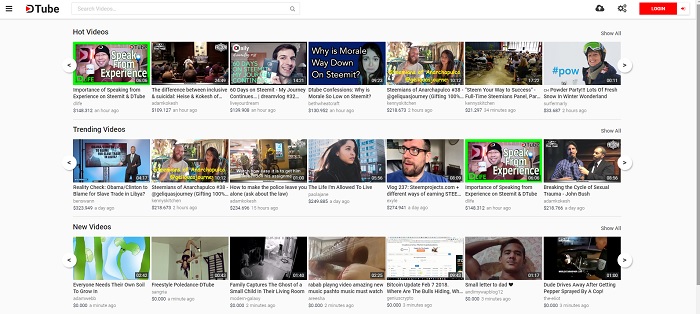The image depicts the DTube homepage, characterized by its distinct, stylized 'D' logo followed by the word 'Tube' in black font. At the top of the page is a search bar, flanked on the right by what appears to be a blurry red button, likely reading 'Login'. The main content area is organized into three horizontal sections, each containing seven video thumbnails arranged in a row.

In the first row, under the section titled 'Hot Videos,' the most prominent thumbnail on the left features a video titled "Speak from Experience," which is uniquely highlighted with a green border. Other videos in this row are less discernible due to poor resolution.

The second row, labeled 'Trending Videos,' contains a middle thumbnail that is slightly more readable, displaying the title "60 Days on something - My Journey Continues," and another that mentions "Why is Morale Way Down on Steemit?" emphasizing the platform's focus on Steemit-related content. There's also a video titled "#POW," but details on other thumbnails remain unclear.

The third section, designated 'New Videos,' is even harder to decipher, with text and thumbnails rendered illegible due to the image's low quality. Despite these challenges, the layout and structure of the DTube interface are evident, showcasing a user-friendly organization of video content into distinct categories.